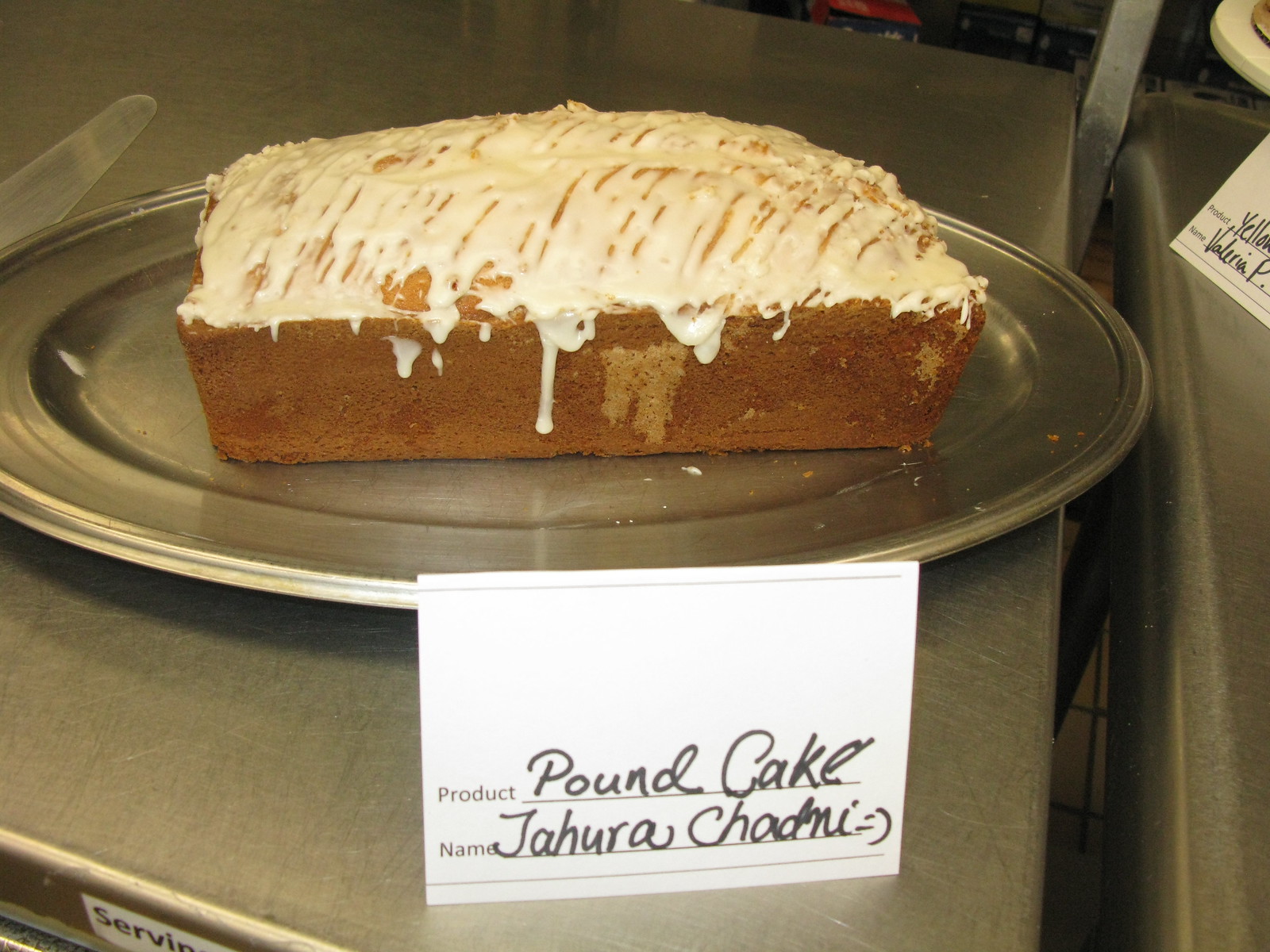Displayed on an oval-shaped silver platter at a bakery counter is a brown pound cake topped with white frosting, reminiscent of a homemade treat baked in a pan with slightly curved top edges. In front of the cake, a neatly printed white label reads "Product: Pound Cake" and "Name: Jahura Chadmi," with a smiley face beside the name. Partially visible next to it is another label for a different product, showing only the word "yellow" and the name "Valeria P." The scene, characterized by hues of brown, grayish silver, and white, suggests a well-organized, boutique bakery setting, likely offering a variety of such freshly baked goods.